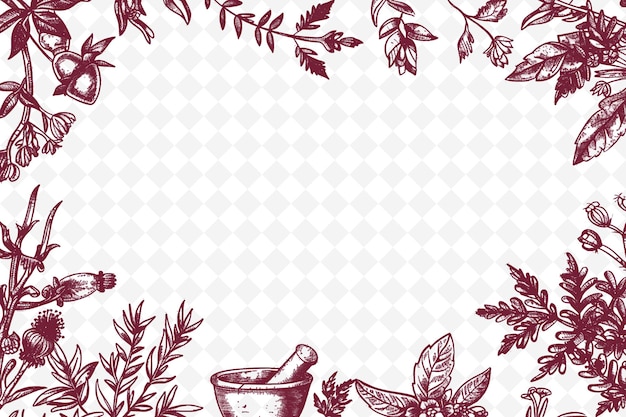The image is a decorative border template featuring a detailed, floral design. The center background consists of white and gray checkered diamonds, which are not intentional and should be transparent. The border surrounding the center is adorned with lush, intricate floral patterns showcasing a variety of red flowers and foliage. At the very bottom center, there is a mortar and pestle; the bowl and stick are outlined in red, traditionally used to grind herbs or other substances. To the left of this mortar and pestle, twigs with small leaves are depicted, while to the right, there is a bulbous flower with black filaments. Above and slightly to the right, a red-stemmed flower with tiny, curved leaves can be seen, alongside an acorn attached to it. The overall ambiance of the border suggests a rich, herbal, and botanical motif, with additional features like thistles on either side and various leaves and floral elements in red and purple hues.